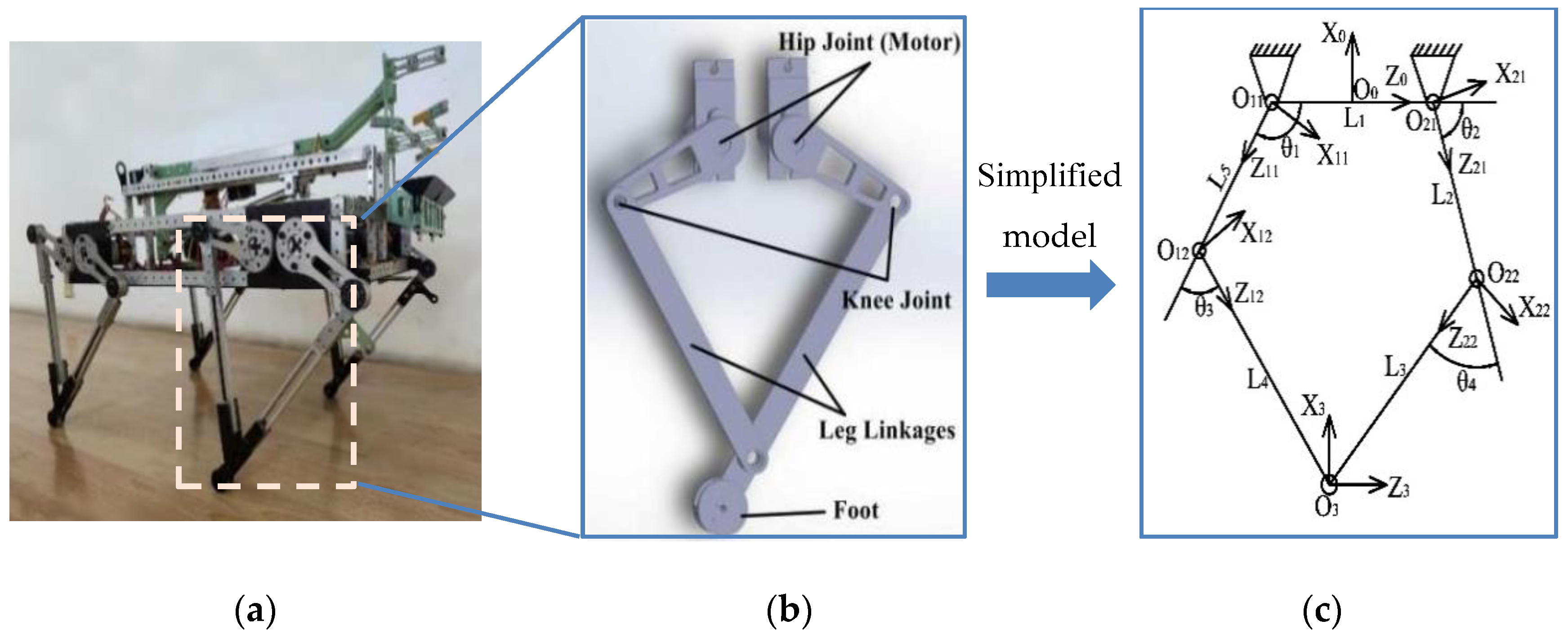The image displays a three-part diagram labeled A, B, and C, showcasing the design of a parallel quadruped robot based on a novel intelligent control system. Part A features a full view of the robotic apparatus resting on a shiny, medium tan hardwood floor, with a dotted line rectangle highlighting the bottom part of its hip joint. Part B zooms in on this highlighted area, detailing the mechanical components with labeled arrows pointing to the hip joint, motor, knee joint, leg linkages, and foot. Part C presents a schematic, simplified model of the robot with a diamond and triangular shapes annotated with letters and numbers, including X, Z, X12, Z12, 03, and 04, explaining the mechanical and control aspects of the design.